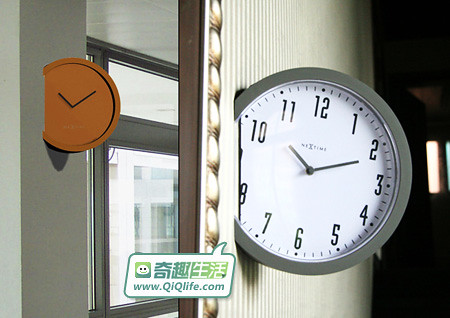The image appears to be a digitally altered or AI-generated composition featuring two distinct clock designs set against different backgrounds. On the left side of the image, there's a gray wall with a window frame through which the outside of a building with multiple windows can be seen in clear detail. Partially embedded into this gray wall is a reddish-brown circular clock face that displays only its hands, positioned at approximately 10:10, with no numbers to mark the hours.

To the right, the wall changes to a design with vertical gray stripes. Mounted on this wall is a larger, more traditional gray-rimmed clock face that displays the numbers 1 through 12, each separated by four small lines indicating the minutes. This clock features an hour, minute, and second hand, and includes the phrase "Next Time" on its face. 

Additionally, in the background on the right-hand side, there is a black area with a small speech bubble graphic. Inside the speech bubble, the text "www.QIQLIFE.com" is prominently displayed, accompanied by Asian characters above it and a smiley face at the end.